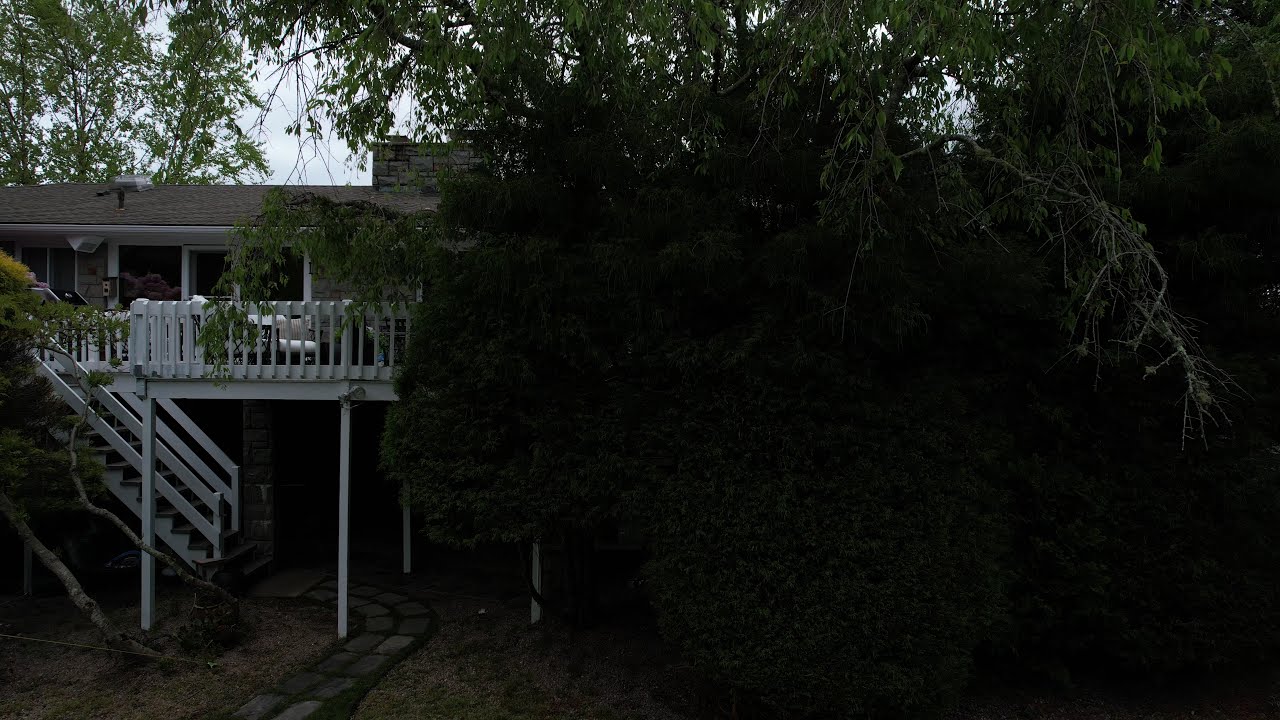The image depicts a residential setting with a single-family home on the left and dense vegetation on the right. The home's elevated white porch is about 10 feet off the ground, supported by thin wooden columns, and features white trim around its windows and sliding doors. A concrete paver walkway and dirt area lie beneath the porch. The house structure appears to be made of concrete blocks, and its roof is tan with a visible chimney. The right side of the image is heavily shadowed due to the camera's exposure settings, making the vegetation appear almost black towards the bottom right corner. However, the greenery hanging from the top is clearly visible and vibrant. The sky is clear, indicating it's daytime. A large, low-hanging tree on the right frames the scene, filling that side of the image with abundant foliage that contrasts against the brightness of the house.